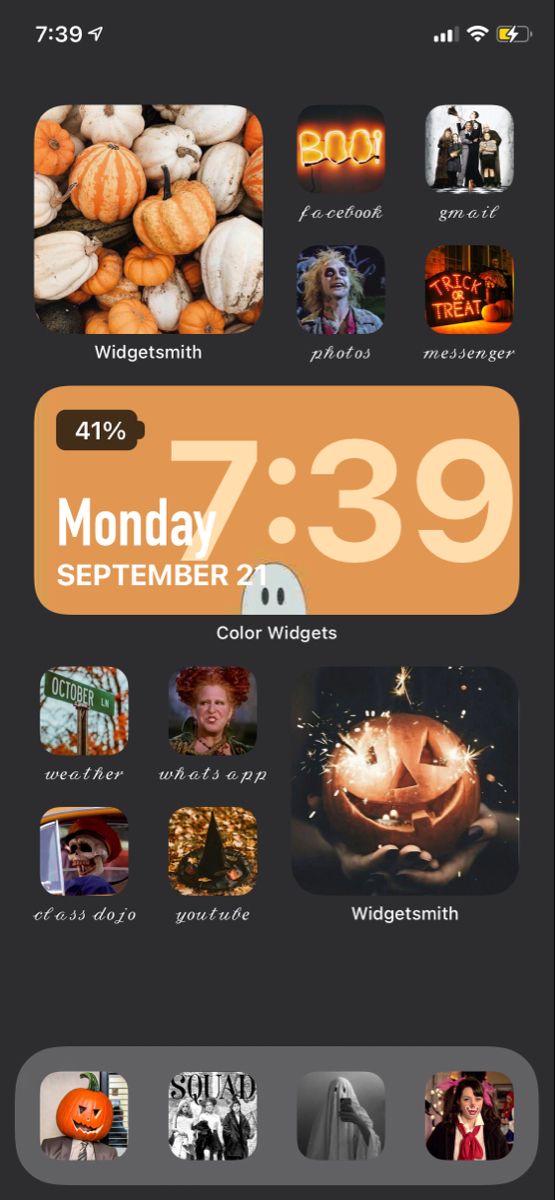This is a detailed screenshot of a mobile phone's home screen. In the top left corner, the current time is displayed. In the top right corner, there are three status icons: the network coverage showing three out of four bars, the Wi-Fi signal displaying full strength with three bars, and an indicator that the phone is currently charging. The screen features a variety of squares and rectangles representing different widgets and app icons.

Central to the display is a prominent rectangular widget showing the current time, day, and date in large text. Below this information is the label "Color Widgets." In the top left corner of the screen, there is a sizeable square widget, approximately the size of four smaller icons, labeled "Widget Smith." This widget features a collection of colorful pumpkins, aligning with a Halloween theme that pervades the screen. Directly below it is a photo widget labeled "Photos," displaying an image of the Beetlejuice character. This Halloween motif ties together the visual elements of the home screen.